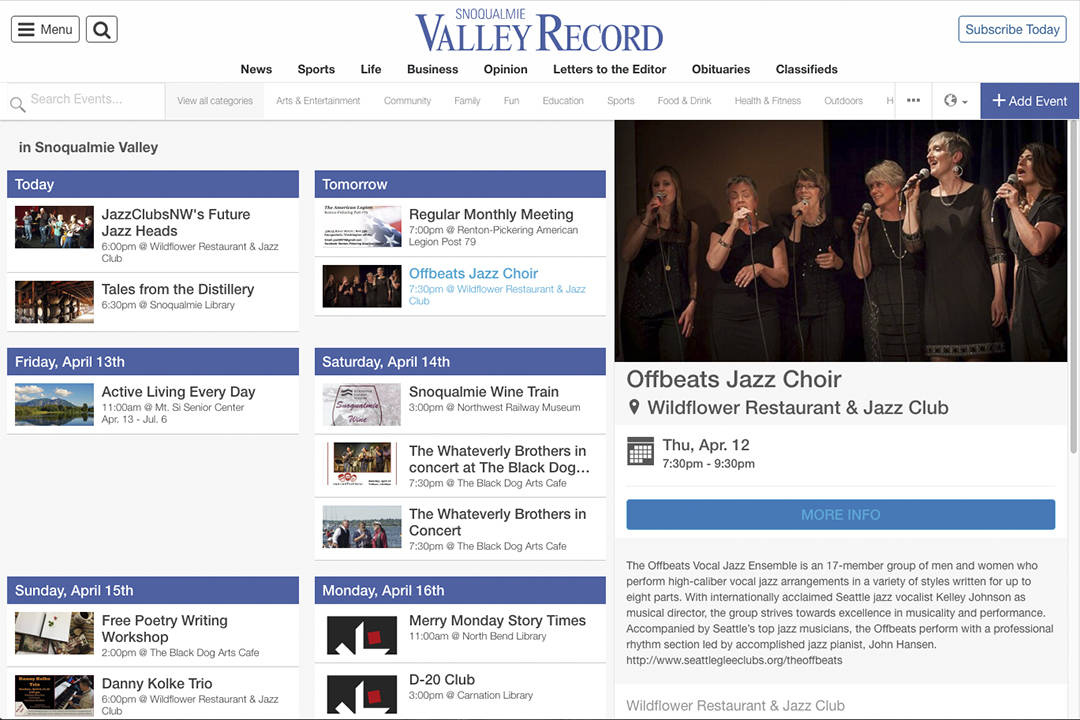This image features a solid white background with various elements arranged prominently. At the center, blue text reads "Snoqualmie Valley Record." The website interface includes several features: 

- In the upper left corner, there is a menu icon and a magnifying glass button for search functionality.
- The upper right corner hosts a "Subscribe Today" button.

Below the header, a horizontal navigation menu displays the following categories in bold black text: News, Sports, Life, Business, Opinion, Letters to the Editor, Obituaries, and Classifieds. 

Under this menu, in light gray text, there is a search bar labeled "Search events" followed by options to view various categories such as Arts & Entertainment, Community, Family Fun, Education, Sports, Food & Drink, Health & Fitness, and Outdoors. To the right of these options is a blue action button labeled "Add Event."

Further down, a color photograph captures the attention. The image showcases six women, all dressed in dark dresses, each holding a microphone. They appear to be in the middle of a performance, given their singing poses and open mouths. The caption below the photo identifies the group as "Off Beats Jazz Choir."